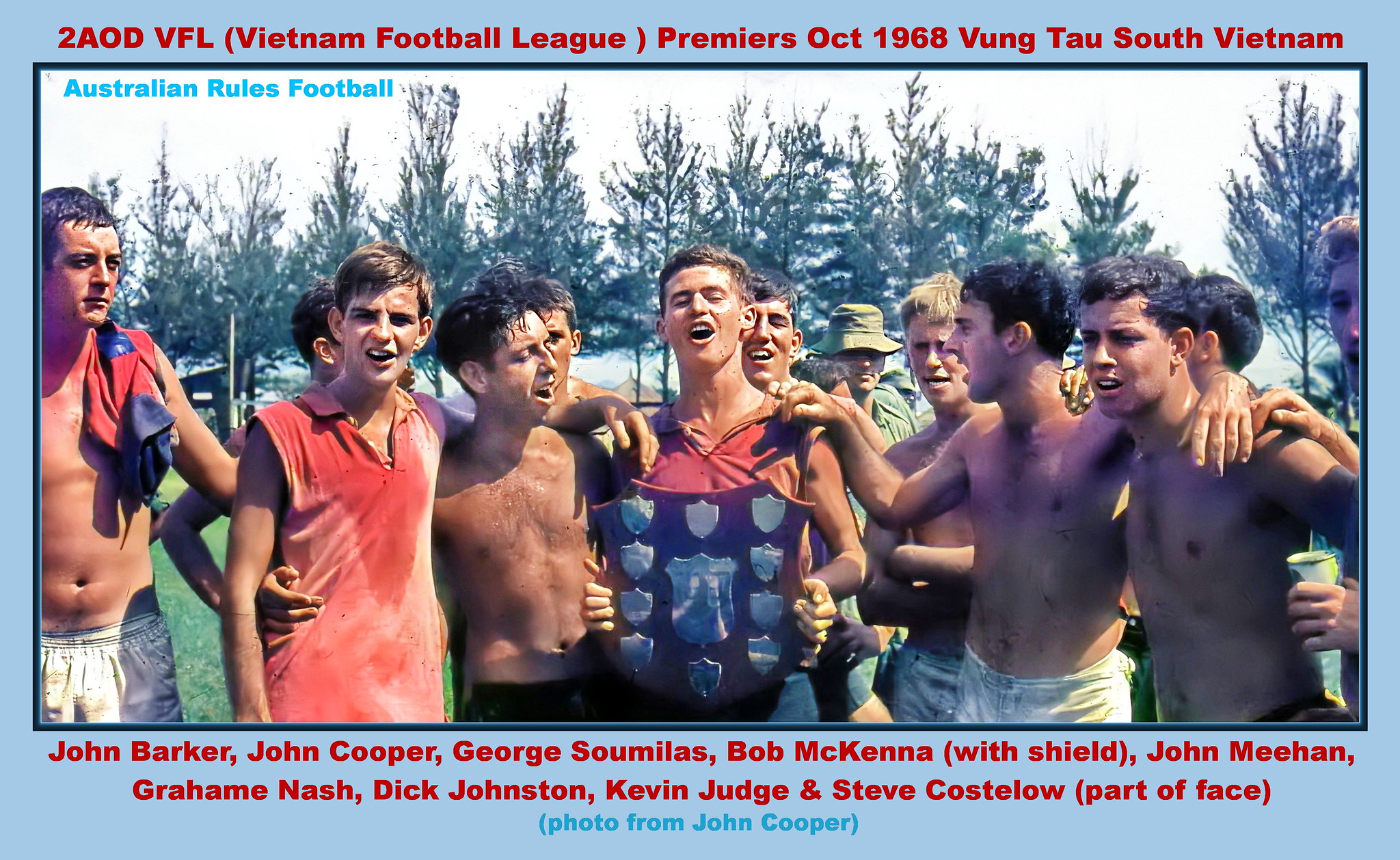This is a wide rectangular color photograph displayed in a digital frame, which is thinner on the left and right sides and thicker at the top and bottom. The frame has a light blue color at the top and a shiny darker blue inner frame. At the top, in bright red font, the text reads "2AOD VFL Vietnam Football League Premieres October 1968 Vung Tau, South Vietnam." Below the image, the text in red lists names: "John Barker, John Cooper, George Soumilas, Bob McKenna (with shield), John Meehan, Graham Nash, Dick Johnston, Kevin Judge, and Steve Costello (part of face)." Further below, in blue text, it reads, "Photo from John Cooper."

The photograph itself captures a group of young men standing outdoors, mostly shirtless while a few wear red sleeveless shirts. They are sweaty, indicating recent physical exertion, perhaps from a football (soccer) match. The central figure, presumably Bob McKenna, proudly holds a wooden shield adorned with glossy metal pieces, signifying an award or trophy. The group stands together with tall leafy trees in the background, and one man in a military uniform—green cap and fatigue style shirt—can be seen among them, reinforcing the image's historical context in South Vietnam during 1968.